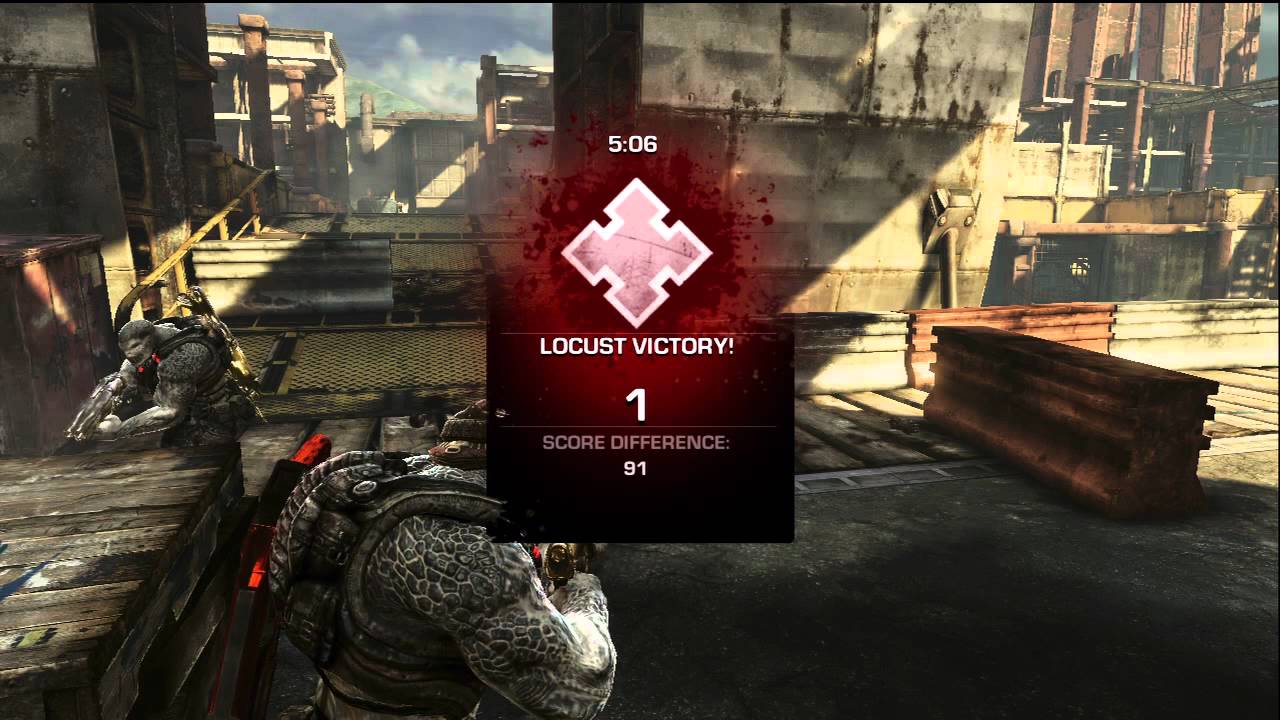The image portrays a scene from a violent shooting video game set in a dilapidated construction site. Two heavily armored men, both wearing grey uniforms and masks, dominate the scene. One character, highlighted near the left, has bulging arm muscles and an imposing stature, while the other is positioned at the front. Both are actively engaged, aiming their guns at an unseen target. The construction site is rusted and deteriorated, providing a rugged backdrop that opens up to an overcast sky. Central to the image is a grim, blood-red label, splattered at the top, displaying "5:06" in white lettering followed by a diamond-shaped icon. Below this, it says "Locust Victory!" with the number "1" and a score difference of "91." The overall atmosphere suggests intense combat and a desperate struggle for dominance.